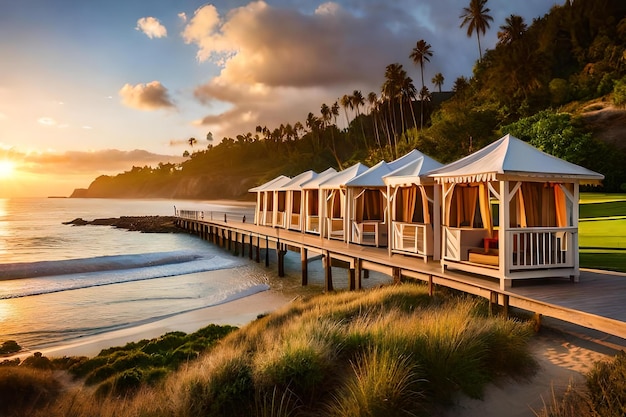The detailed, cleaned-up caption for the image is:

The scene captures a serene, tropical setting at either sunrise or sunset, rendered in full-color and horizontally rectangular without specific borders. A tranquil beach with soft, slow waves stretches across the bottom, bordered by tall grasses and pristine white sand. Above the beach, a meticulously manicured strip of bright lime-green grass evokes the manicured lawns of a golf course. The landscape is dotted with palm trees, with more visible off in the distance.

A well-crafted wooden pier extends into the shimmering water, populated by a row of seven to nine identical white-roofed cabanas or bungalows, aligned in a vertical row from the right center to just left of center. Each cabana is enclosed with wooden posts and fencing, possibly with optional curtains for privacy, and features interior seating arrangements for visitors to relax and enjoy the view. The roofs and exteriors of the cabanas are white, complemented by hints of tan and orange.

In the background, the sky transitions from vibrant blue to a rich palette of orange, hinting at either the rising or setting sun. Heavy clouds tinged with gray and purple add to the dramatic atmosphere. A verdant peninsula extends into the water, adorned with clusters of lush greenery and tall palm trees, enhancing the tropical escapism of the scene. Overall, the peaceful, painterly quality of this photograph evokes an image ideal for display in a tranquil, inviting space such as a hotel.